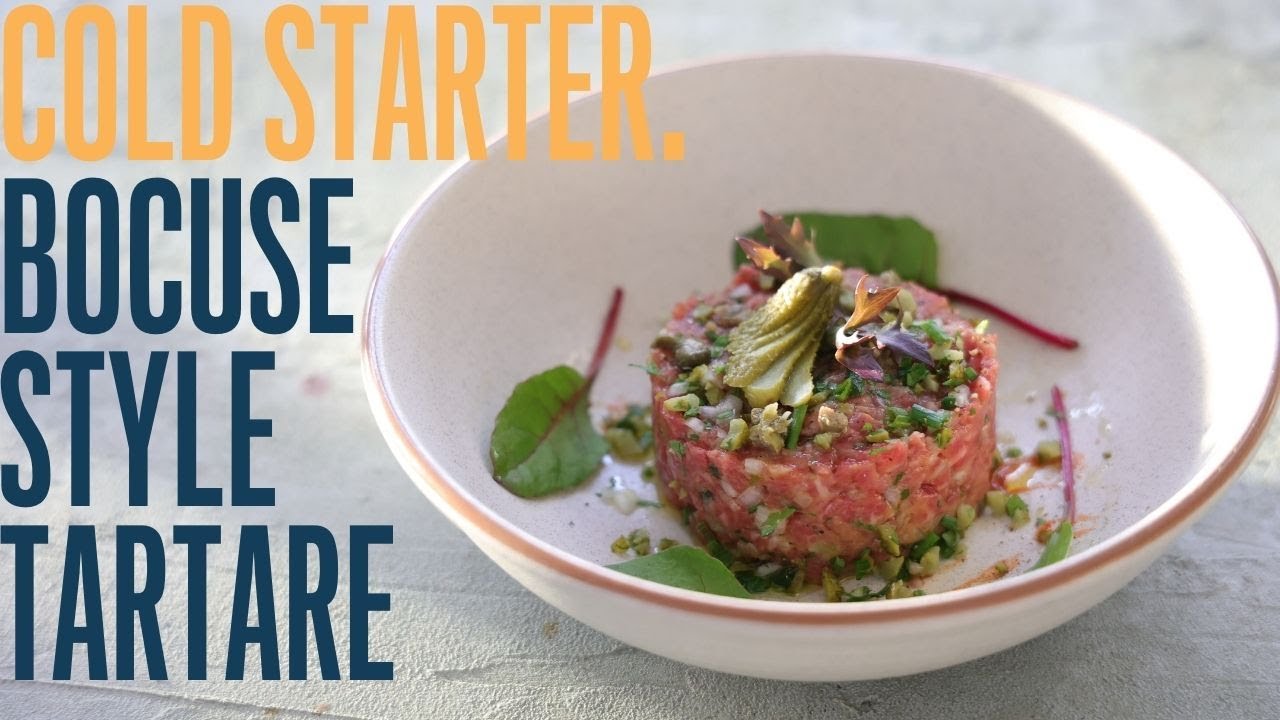The image features an elegant advertisement showcasing a Cold Starter Bocuse Style Tartare. Central to the photo is a pristine white bowl with a distinct terracotta rim, sitting on a white countertop. Inside, a hockey puck-sized round of raw beef tartare takes center stage, mixed with finely diced onions, tomatoes, and herbs. This exquisite dish is topped with fresh slices of avocado and garnished with arugula leaves, green foliage with red stems, and a delicate scattering of additional herbs. The visually pleasing arrangement highlights the dish's gourmet appeal. To the left of the bowl, the text "Cold Starter" appears in large, bold yellow letters, while "Bocuse Style Tartare" is displayed below in a striking dark blue font.